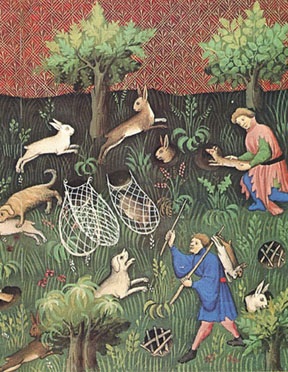This detailed medieval-style illustration, possibly from the 13th or 14th century and perhaps part of a tapestry, depicts an intense rabbit hunt under a textured red wine-colored sky. The scene is set in a lightly forested area with scattered trees and ground covered in grass and small plants. Two men, both dressed in medieval gowns, are hunting rabbits. The man in the foreground wears a blue robe and blue leggings, carrying a pole with two dead rabbits and a stick in his right hand, while a white dog leaps in front of him. The other man, positioned at the top right, is clad in a reddish-salmon-colored robe and white leggings, kneeling with an old-fashioned cap on his head. He appears to be checking and setting traps. Various rabbits are depicted throughout the image: one white rabbit and one larger brown rabbit are leaping near the trees; others are being caught in wooden traps covering their burrows or ensnared in white nets. Hunting dogs are actively participating, with one dog visibly on top of a rabbit and another in the process of catching one. The overall composition captures the dynamic and chaotic nature of the hunt amidst a vividly colored landscape.